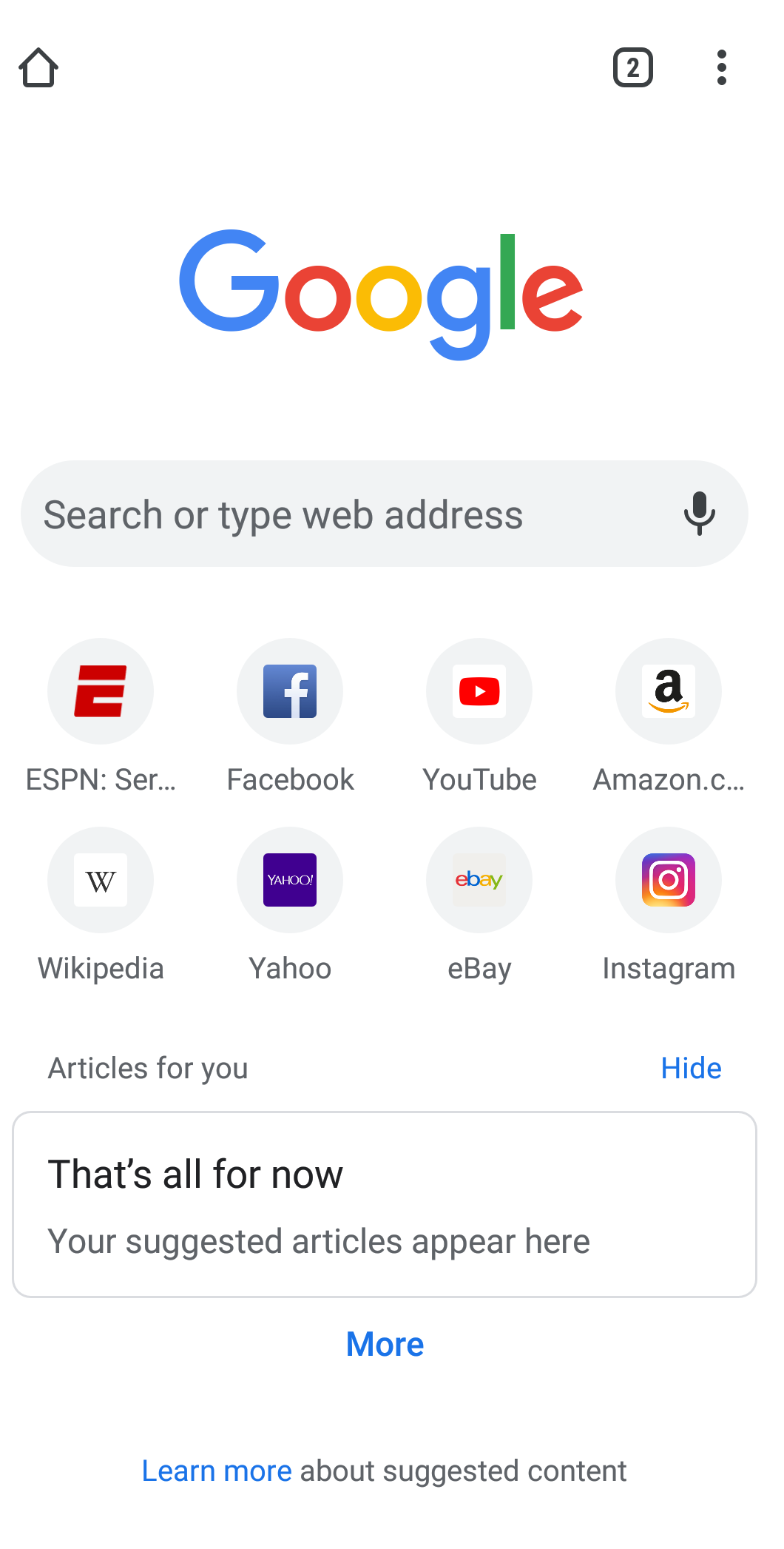This image appears to be a vertically oriented screenshot taken from a mobile device, possibly an Android or iPhone. 

At the top of the screen, there is a large white area featuring navigation symbols. On the upper left, a black arrow points upwards, and on the upper right, there is a black-rimmed rectangle with the number "2" inside. Adjacent to this are three vertical black dots. Below this navigation area, we see the Google logo: a capital "G" in blue, followed by lowercase letters: a red "O", a yellow "O", a blue "G", a green "L", and a red "E". 

Directly under the Google logo is a grey oval search bar with the text "Search or type web address" in black, and a microphone icon on the far right.

Beneath the search bar, there are two rows of app icons organized in sets of four:

- The first row includes:
  1. A red "E" with "ESPN" partially visible.
  2. A grey circle with a blue Facebook icon and the text "facebook".
  3. A grey circle with the red and white YouTube icon and the text "YouTube".
  4. A grey circle with the Amazon logo (a black "A" with a gold smile) and the text "Amazon.com".

- The second row features:
  1. A grey circle with a white "W" and the text "Wikipedia".
  2. A grey circle with a purple square containing white letters "Yahoo" and the text "Yahoo".
  3. A grey circle with the eBay logo and the text "eBay".
  4. A grey circle with the Instagram logo and the text "Instagram".

Below these app icons, there is a section labeled "Articles for you" in black letters on the left, with the option to "Hide" in blue letters on the right.

Following this, there is a light grey box with the text "That's all for now" in black and a subtitle in a fainter black that reads "Your suggested articles appear here".

At the very bottom of the screen, text options are visible in blue and black:
- "More" in blue letters.
- "Learn more" in blue letters.
- "About suggested content" in black letters.